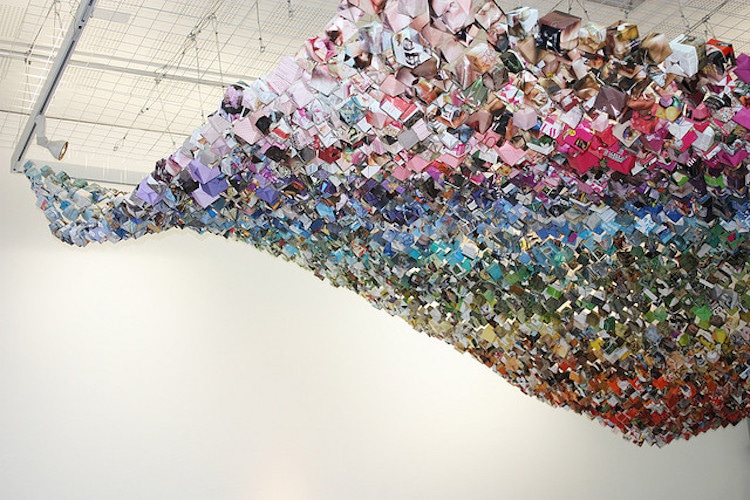The image depicts an intricate artistic installation that is likely displayed in a museum or at a high-profile event. The artwork is suspended from a complex array of metal bars and wires fastened to the white ceiling. The setup includes additional wires and strings, along with a spotlight on the left side, strategically illuminating the piece. The installation features a cascade of multi-colored cubes, each with its distinct image, collectively forming a stunning, rainbow-like wave that starts narrow at the top and expands as it descends. The colors in this wave transition smoothly through a spectrum of red, orange, yellow, green, blue, pink, and finally white at the bottom, creating an optical effect that appears more cohesive and striking when viewed from a distance. The scene is set against pristine white walls, enhancing the vibrant colors and geometric precision of the artwork, giving it the illusion of growth as it approaches the floor.